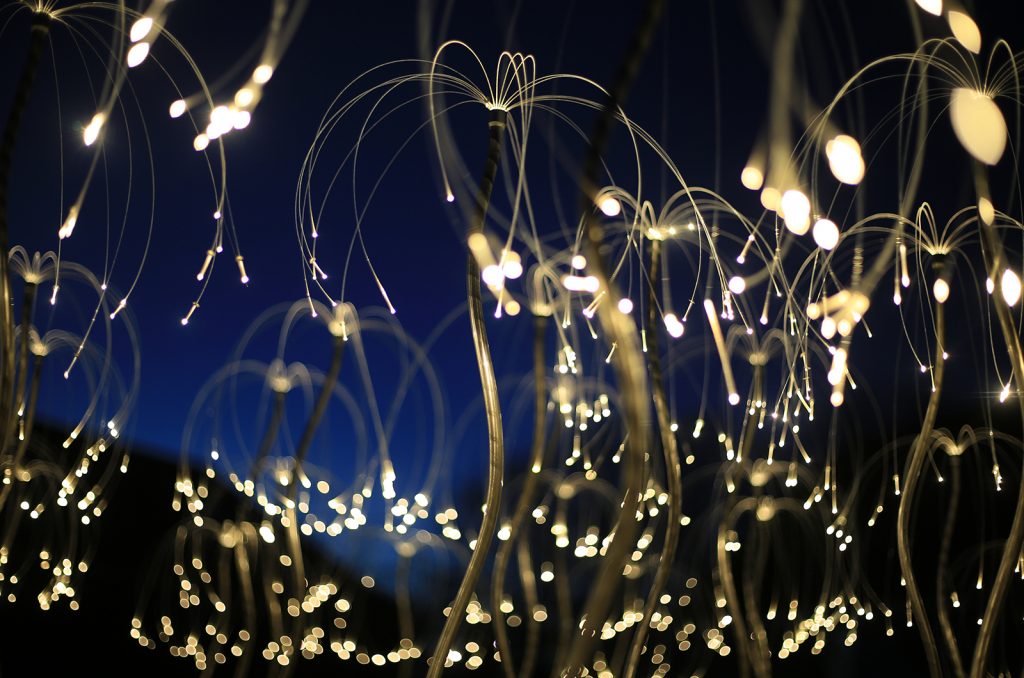The horizontal rectangular image displays a mesmerizing nighttime scene that captures the interplay of light and shadow. The backdrop is a dark blue sky transitioning to black as it nears the horizon, suggesting a late or twilight hour. In the foreground, numerous illuminated objects rise up resembling either whimsically arranged fairy lights, fiber cables, or possibly metallic plant-like structures. These structures are anchored in the ground, emerging like the stems of plants and branching out in all directions. The lights at their tips exude a soft, enchanting glow reminiscent of Christmas light bulbs or fireflies. The blurriness of the image imbues it with a dreamy quality, making the scene appear busy yet harmonious, and evoking the sensation of a magical fountain of light against a serene dark sky. The overall impression is one of ethereal beauty, combining elements of both natural and man-made aesthetics.